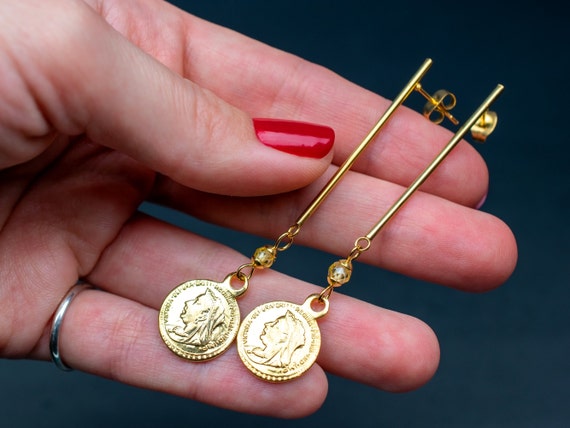A woman's left hand, adorned with a silver pinky ring, is elegantly holding a pair of gold earrings. Her crimson red nails, especially the prominent thumbnail, stand out against her skin. In the image, her hand is oriented with the palm on the left and fingers extending to the right. The earrings, each featuring a long, slender gold rod almost spanning the length of her pinky finger, rest along her index and middle fingers. These gold rods lead down to intricate components: a small gold bauble connected to a ring, which in turn attaches to a gold coin pendant. Each pendant showcases a female figure, likely Queen Victoria, gazing to the left. The coins are slightly smaller than an American quarter and add a touch of antiquity to the elegant earrings. The post and butterfly backing of the earrings are also visible, emphasizing their detailed craftsmanship.